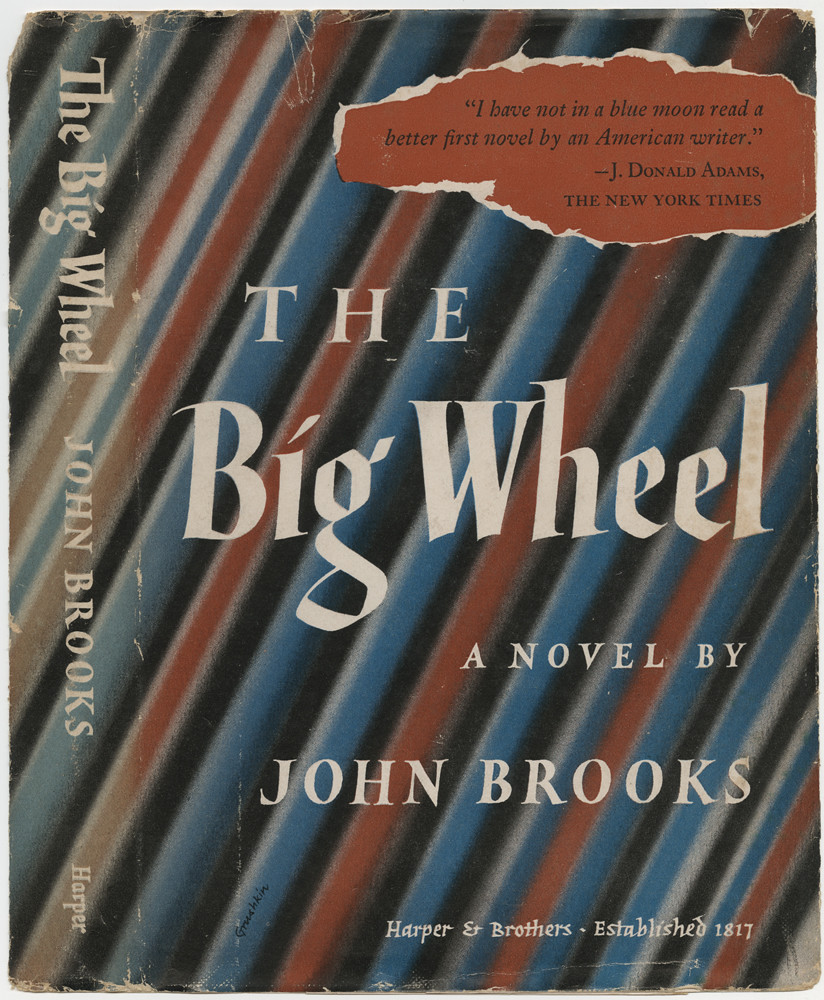This image depicts the cover of a very old and weathered paperback book titled "The Big Wheel" by John Brooks, published by Harper and Brothers, established in 1817. The cover exhibits significant signs of wear, including frayed and ripped corners, as well as a tattered binding, suggesting heavy use over time. The spine visible on the left side reads, "The Big Wheel, John Brooks, Harper." The cover features a diagonal striped pattern with recurring colors of black, light red, blue, and white. Notably, the design includes a section at the top featuring a white, torn-paper effect with a red background and black text containing a quotation: "I have not in a blue moon read a better first novel by an American writer," attributed to J. Donald Adams of The New York Times. The main text across the center of the front cover prominently displays, "The Big Wheel, a novel by John Brooks," with the publisher's name and establishment date at the bottom. This detailed and characteristic design highlights the book's classic and time-worn appearance.